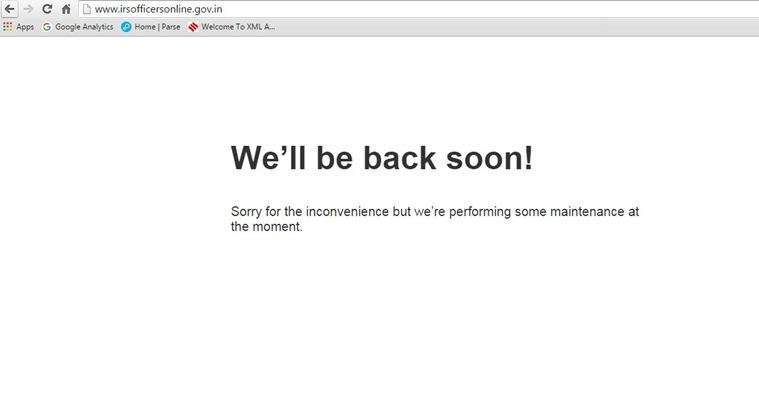The image appears to be a screenshot of a computer screen. Dominating the center of the screen is a prominent message in large black letters stating, "We'll be back soon!" Directly below this, in smaller text, is a note of apology: "Sorry for the inconvenience, but we're performing some maintenance at the moment."

At the top of the screen, a white address bar is visible displaying the URL: www.irsofficeofficersonline.gov.in. Accompanying this are several icons and labels. There is a grid of nine dots adjacent to the word "Apps," followed by the colorful "G" logo for Google, labeled "Google Analytics." Additionally, there is a blue circle with a symbol inside, labeled "Home," followed by "PARSE." Another icon, a square made up of three red lines within a white square, is labeled "Welcome to XML." Lastly, there is an icon starting with "A" followed by three dots.

This screenshot seems to announce a temporary website maintenance and shows the typical navigation and service icons you might find on such a page.